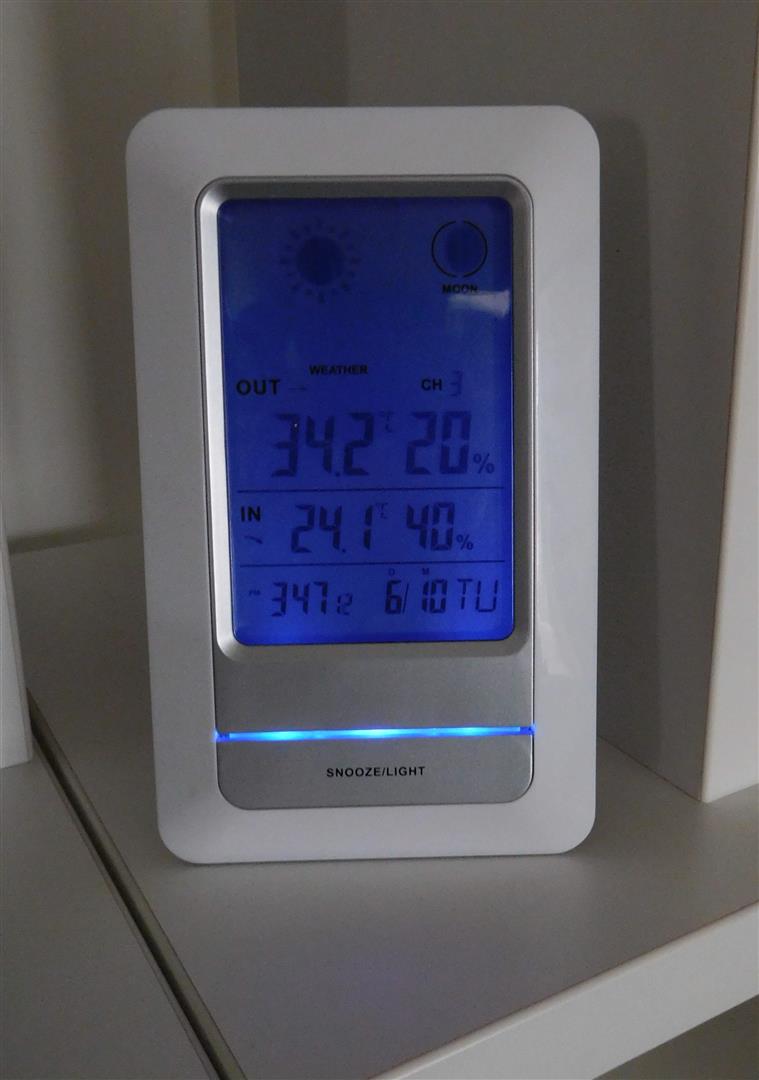This vertical image showcases a close-up of a white plastic device labelled as a "snooze/light." The device features a blue screen at its upper center displaying black digital readouts divided into three rows. Due to dim lighting, the labels for these rows are difficult to discern. The first row on the right reads "34.2" and "20%," while the second row centrally displays "21.4" and "40%." The smaller third row lists "34.7," "6," "10," and "TU," the latter likely indicating Tuesday, with the time showing as "6:10." Above the device's name is a lighter grayish insert containing a thin, illuminated bar extending horizontally in a bluish-green light. The device rests on a thick plastic shelf, and the background consists of what appears to be white plastic walls, suggesting the setting is inside a cabinet or on a shelf.